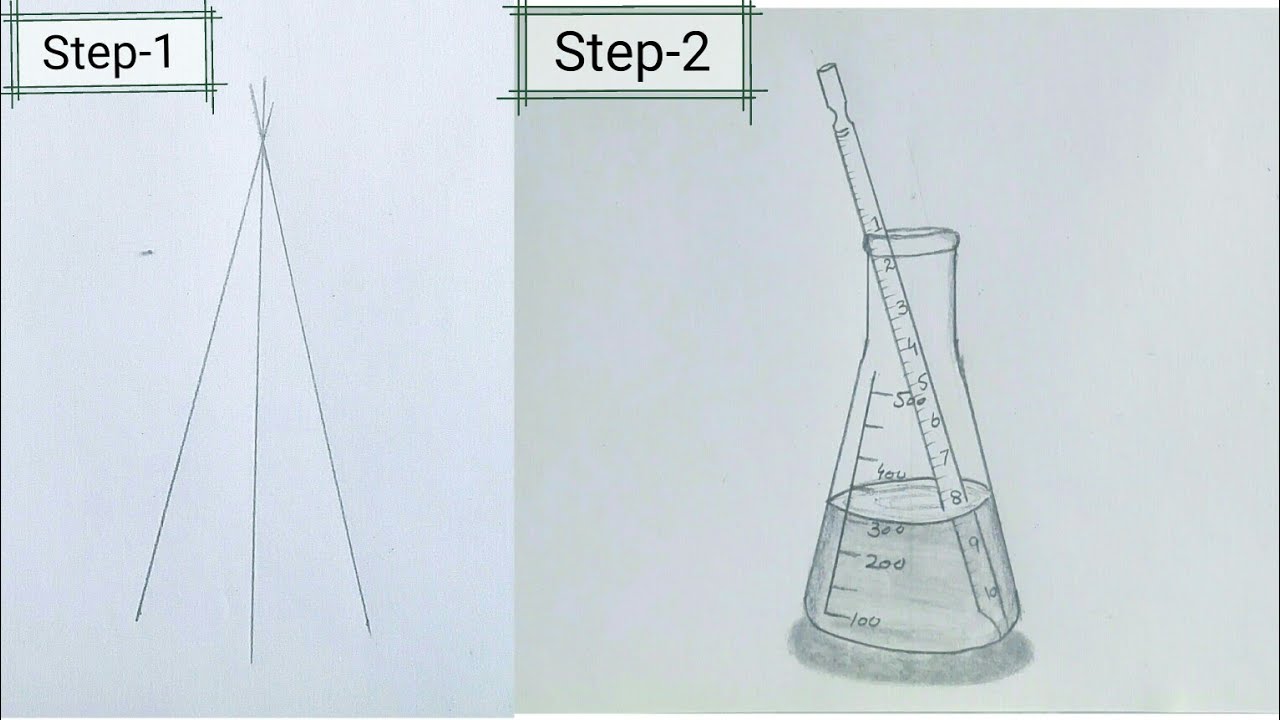The image depicts a step-by-step tutorial on drawing an Erlenmeyer flask with a graduated pipette inside it, shown across two steps on plain white paper. Step 1, positioned on the left and outlined by green lines, introduces the initial sketch: a basic wireframe consisting of three intersecting lines forming a triangular base, resembling a teepee structure. Step 2, found on the right and similarly outlined, presents a completed drawing of an Erlenmeyer flask with a narrow top that broadens out into a conical shape. Inside the flask is a graduated pipette, erroneously referred to as a thermometer in one description, measuring liquid levels up to 300 milliliters. The flask itself is marked with measurements ranging from 100 to 500 milliliters. This second step elaborates on the complexity, showcasing the fully realized flask partially filled with liquid just above the 300 milliliter mark.